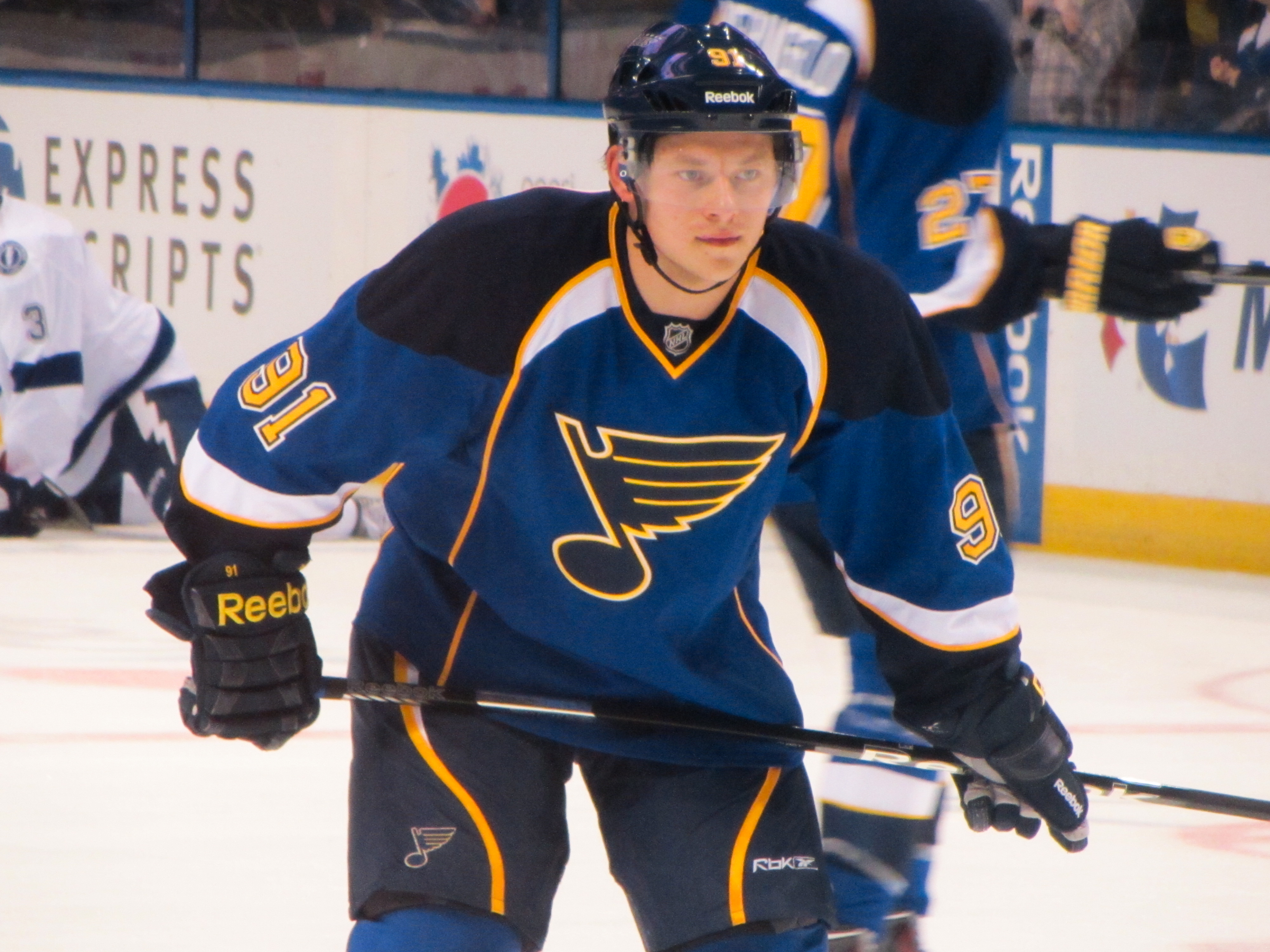In the image, we see a dynamic hockey game in progress featuring teams identified by their distinct uniforms. The St. Louis Blues players are prominently depicted wearing navy blue jerseys with a lighter blue accent and yellow numbers. The team's logo, resembling a winged music note, is visible on their apparel. Opposing them are the Tampa Bay Lightning players, dressed primarily in white with navy blue details. The rink is pristine white, punctuated by red lines marking the ice. Surrounding the rink is a white barricade featuring the Reebok logo, and transparent glass shields the enthusiastic fans visible in the background. This scene captures the excitement and energy of an NHL match between the St. Louis Blues and the Tampa Bay Lightning.